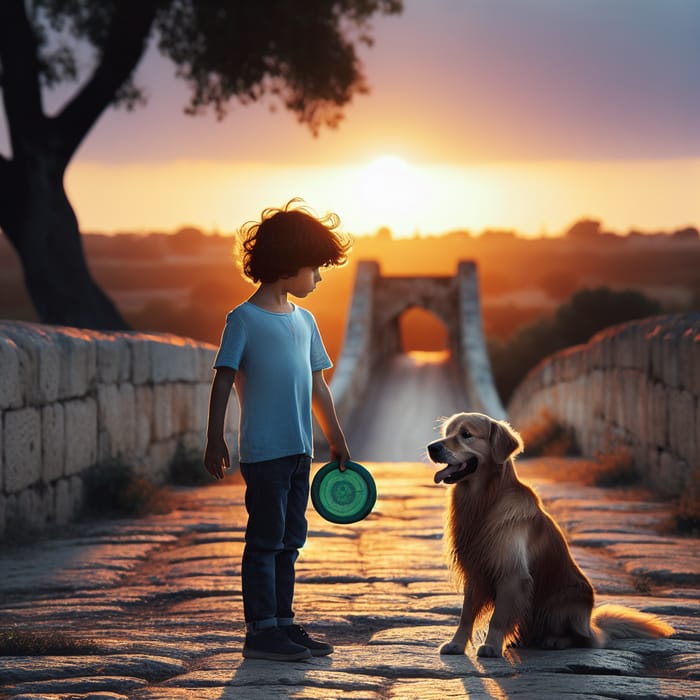The image is an artistic, possibly AI-generated scene, depicting a young boy and a golden retriever on a cobblestone bridge. The bridge, made of stone, arches slightly and extends into the background, creating a sense of depth. Both the boy and the dog are positioned on the bridge, with the boy standing and holding a green frisbee detailed with dark and light green lines. He is dressed in blue jeans, a blue t-shirt, and tennis shoes, his medium-length brown hair slightly messy. The golden retriever, tan with some white accents, is sitting upright on its haunches, mouth open and panting, seemingly awaiting the throw of the frisbee. The boy's gaze is fixed on the dog, while the dog appears to be looking off into the distance. To the left of the scene, there's a silhouette of a tree, and further in the background, the sun is rising, casting a golden glow and illuminating the horizon with bushes and an orange sky that transitions into blue.